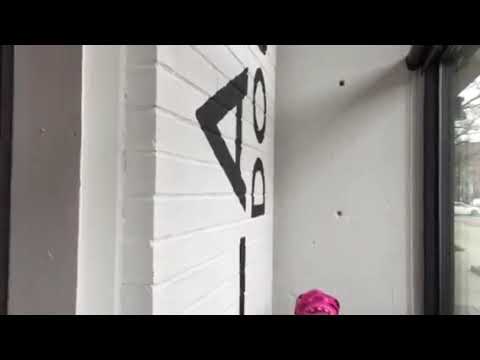This photograph captures an indoor setting featuring a white cement wall in the foreground with two holes. The wall on the left is also painted white but has a black design with lines, which includes sideways black letters "A," "D," and "O." Framing both the top and bottom of the image are two horizontal black strips. To the right, there is a doorway or screen door through which daylight can be seen, indicating an outdoor area. At the bottom center of the image, the top portion of a person's head is visible, distinguished by a fuchsia pink cap. The overall color palette in the photograph includes white, black, gray, silver, dark green, and pink.